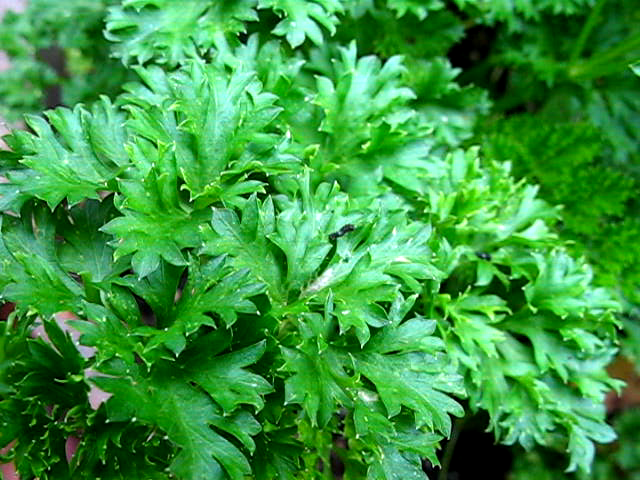This image features a close-up of a vibrant, green, spiky-leaved plant, possibly a type of herb or bush, which dominates the frame. The plant's leaves, resembling those of a holly bush, are characterized by their bright green color, spiky edges, and curved, pointy tips. The leaves appear wet, emphasizing their glossy texture. There are small spikes or nubs along the edges of these leaves. Light reflecting off the right side of the leaves gives them an almost light gray hue. The background, which is mostly blurry, features other green plants and suggests the plant might be in a planter with hints of a brick or tiled floor visible through the foliage. The left bottom corner of the image reveals a reddish-brown object behind the leaves. Additionally, the lack of sharp shadows and directional light indicates an overcast lighting condition, creating a soft and even illumination across the entire plant.